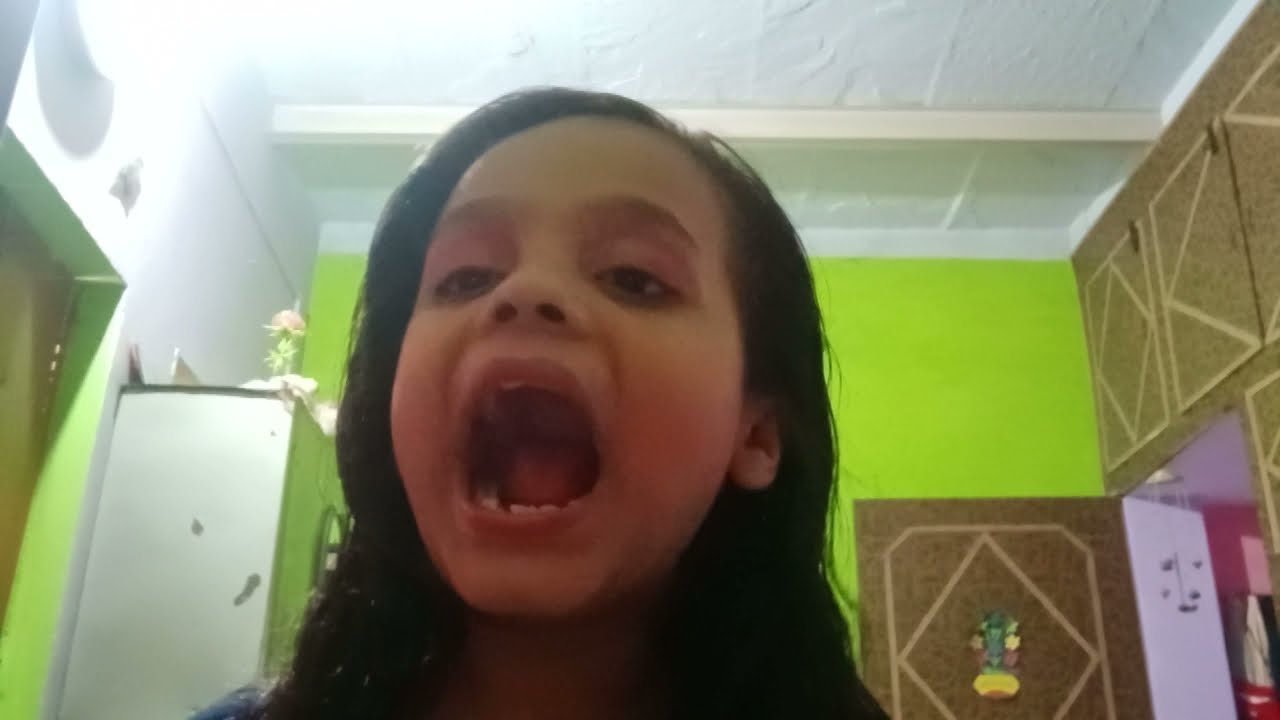A small girl with long, brown hair parted to the side and brown eyes is standing very close to the camera with her mouth open wide, possibly showing where a tooth fell out on the bottom. Her teeth and tongue are clearly visible. Behind her, there is a bright lime green wall. To the left, there's an open door with a silver doorknob, above which hangs a bright light. The ceiling is white with exposed rafters. To the right of the child, an opening appears to lead into another room that looks like a kitchen, featuring some cabinetry, a refrigerator, and a cabinet with a flower and other items on top. A brown wardrobe with open doors displaying a pink wall inside is also visible. The scene is brightly lit and full of vivid colors and details.